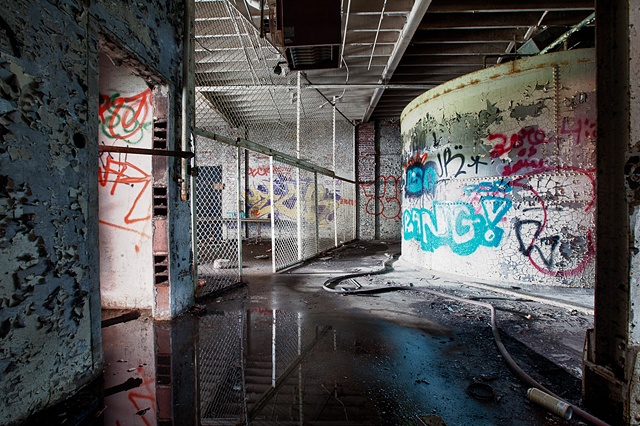The image depicts a grimy and abandoned building with a grungy atmosphere, accentuated by dirt and debris. The space appears to be an underground or enclosed area, possibly a former garage, characterized by its cement construction. The photograph is oriented vertically, capturing multiple rooms. On the left side, there is a wall leading to an open, heavily dilapidated doorway, featuring stagnant pooled water and walls with extensive peeling and distress.

Dominating the middle of the scene is a white chain link fence that extends to the ceiling, implying a separative barrier within the space. Directly behind the fence, sections of the building stand fenced off, potentially resembling a caged area. To the right of the fenced section, a curved wall can be seen, entirely covered in an array of graffiti with various scribbles and spray-painted letters in red, green, and other colors. Another distinguishable blue wall in the forefront further illustrates the prevalent graffiti.

The floor below is muddy and dark gray, scattered with white dust and puddles of water, suggesting either rainwater accumulation or deliberate water spraying. A gray hose stretches from the bottom right of the image to the top, adding to the chaotic and neglected ambiance of the environment.